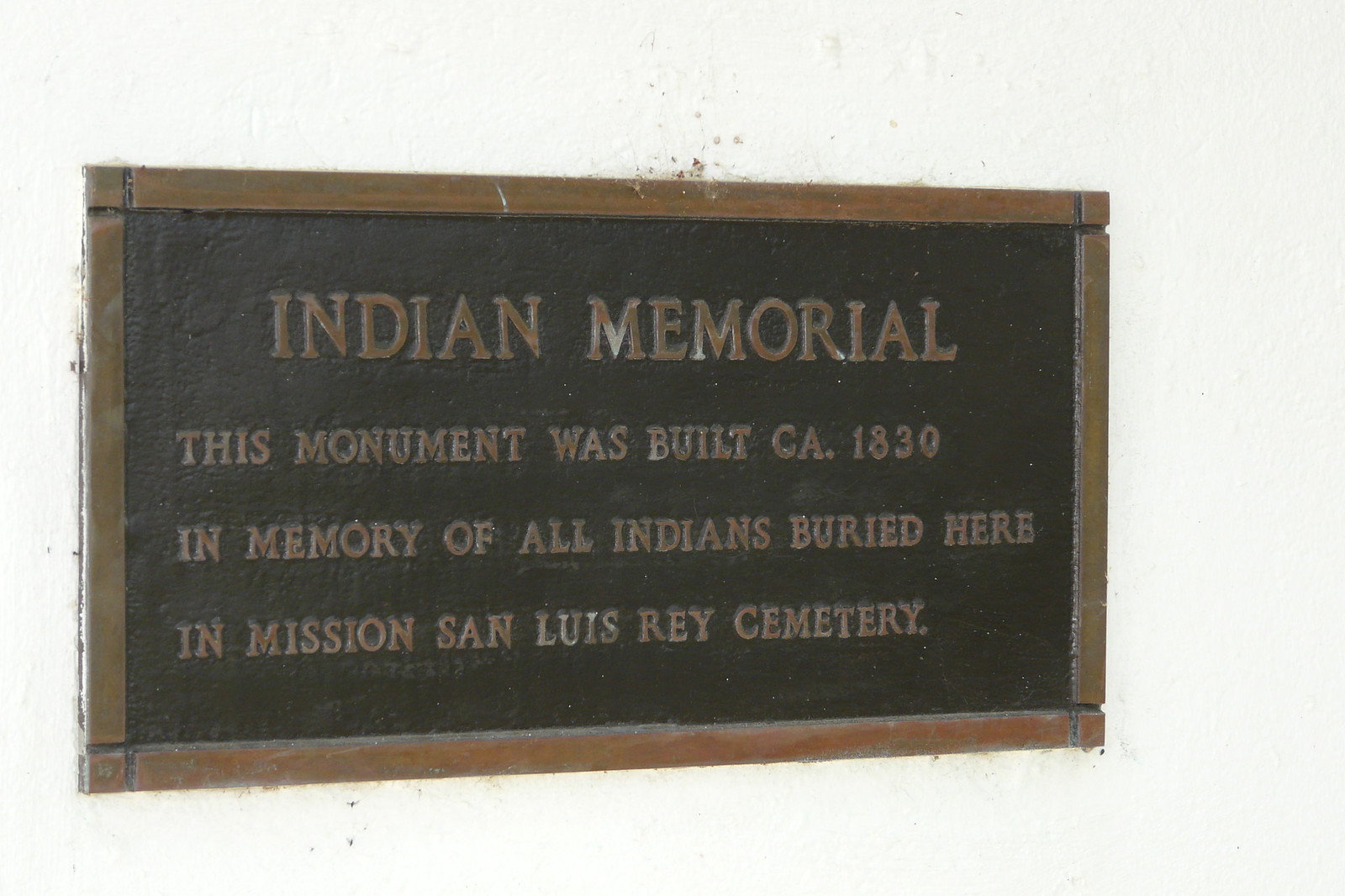The image shows a photograph of a bronze memorial plaque fixed onto a white wall. The plaque features a brown bronze border and a black face with bronze embossed lettering. At the top of the plaque, in large capital letters, is the title "INDIAN MEMORIAL." Beneath the title, in slightly smaller capital letters, the inscription reads: "THIS MONUMENT WAS BUILT C.A. 1830 IN MEMORY OF ALL INDIANS BURIED HERE IN MISSION SAN LUIS RAY CEMETERY." The corners of the memorial plaque are decorated with small decorative squares that are connected by longer lines.